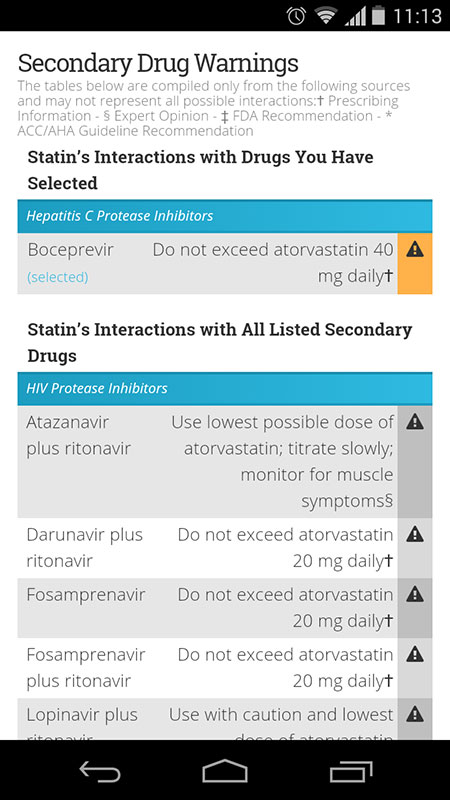The image appears to be a screenshot taken from a mobile phone, as indicated by the black status bar at the top which displays an alarm icon, Wi-Fi signal strength, cellular data bars, battery life, and the current time, noted as 11:13. This screenshot shows a webpage or an application screen containing important medical information about drug interactions.

At the top, in large black letters, the heading reads "Secondary Drug Warnings." Beneath this heading, a disclaimer explains that the tables below are compiled from various authoritative sources, including prescribing information, expert opinion, FDA recommendations, and ACC/AHA guideline recommendations. It also mentions that the tables may not represent all possible interactions.

Following the disclaimer, another prominent heading in a larger font reads "Statins Interactions with Drugs You Have Selected." 

The content is organized into different boxes for better clarity:

1. **Hepatitis C Protease Inhibitors**:
   - This section is highlighted with a blue bar and lists specific medications, including "Boceprevir."
   - There is a directive to "not exceed atorvastatin 40 milligrams daily."
   - Adjacent to each listed medication, there is a yellow warning box featuring a black exclamation point, emphasizing critical caution.

2. **HIV Protease Inhibitors**:
   - This section is also highlighted with a blue bar.
   - It lists five different medications, each accompanied by a similar yellow warning box featuring a black exclamation point, indicating the importance of adhering to the warning information.

At the bottom of the screenshot, there is a black box containing phone icons, suggesting options for navigation or additional actions within the application or website. 

In summary, the image meticulously guides the user through critical information regarding interactions between statins and specific protease inhibitors used in treating Hepatitis C and HIV, with clear visual cues for warnings and restrictions.